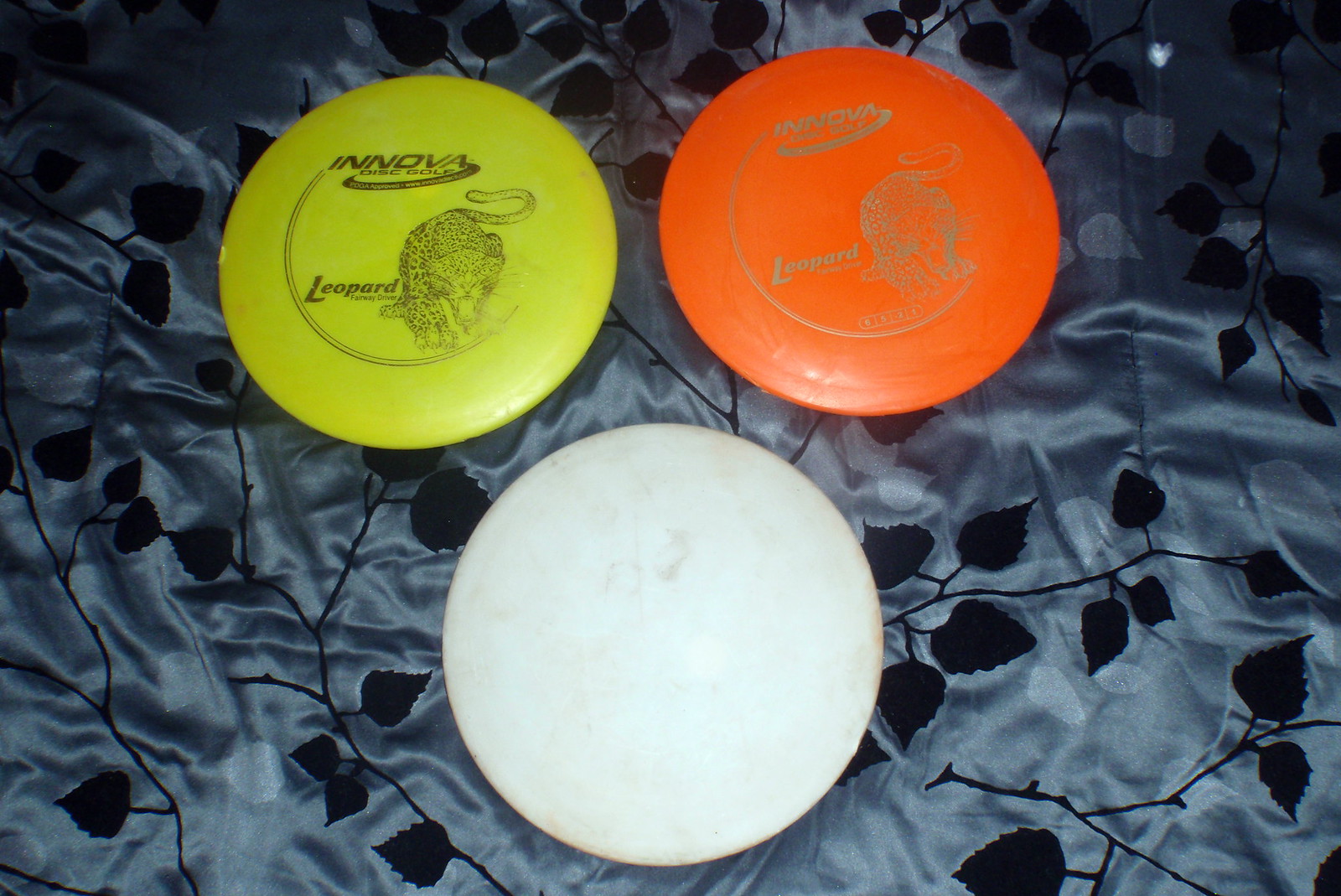The image is a photograph of three frisbees arranged in a triangular formation on a luxurious, satin-like fabric. The fabric is a dusky blue-gray color with an intricate black vine and leaf pattern, appearing silky and crinkled in the light, adding a detailed texture to the scene. The top-left frisbee is a vivid lime green, featuring the words "Innova Disc Golf" at the top and "Leopard Fairway Driver" along with a detailed drawing of a growling leopard on the side. The top-right frisbee is bright orange, bearing the same inscriptions and leopard illustration as the lime green one, though the print is somewhat faded. The bottom-center frisbee is a solid white, with a marbled appearance and looking quite worn, with only faint traces of a once visible logo. The entire setup rests on this ornate fabric, providing a rich backdrop that highlights the unique design and condition of each frisbee.